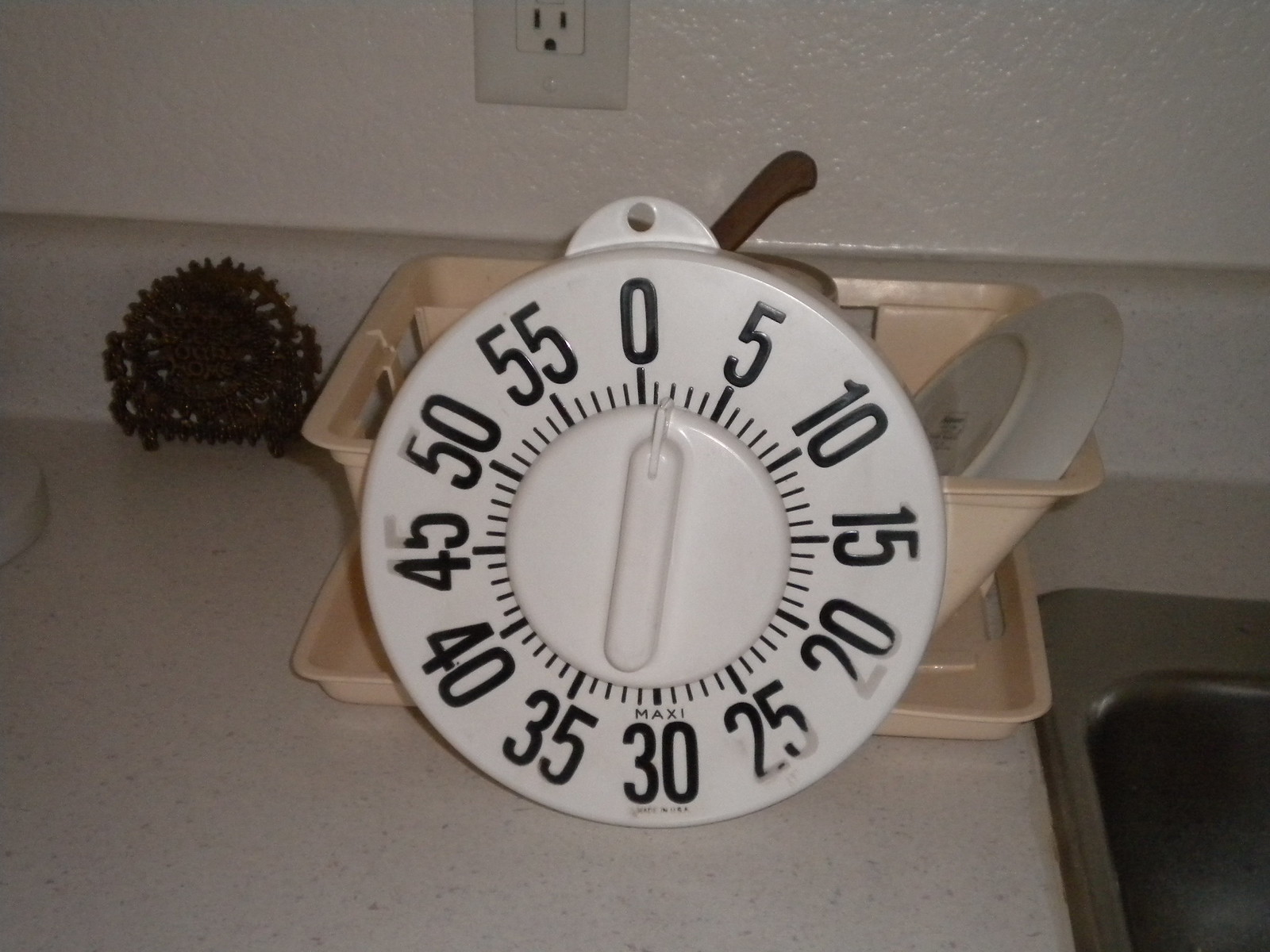This detailed close-up photograph captures an exceptionally large kitchen timer prominently situated on an off-white Formica countertop with grey and black specks. The timer features a round, white face with black numbering and increments of 5, starting at 5 and going up to 55, with 0 positioned at the top center and 30 at the bottom. A central raised dial or crank is used to set the time, and the timer has a small tab with a hole at the top, suggesting it can be hung. The background reveals a beige plastic dish drying rack holding a white plate on the right and a wooden-handled utensil sticking up behind it. To the left of the drying rack sits a decorative metal ornament, possibly bronze or brass. A stainless-steel sink is partially visible in the lower right corner, and a white textured wall frames the upper portion of the image, showcasing part of a power outlet to the upper left. The entire scene is set on a kitchen surface, emphasizing the size and prominence of the kitchen timer which is propped against the dish drying rack, towering over its surroundings.